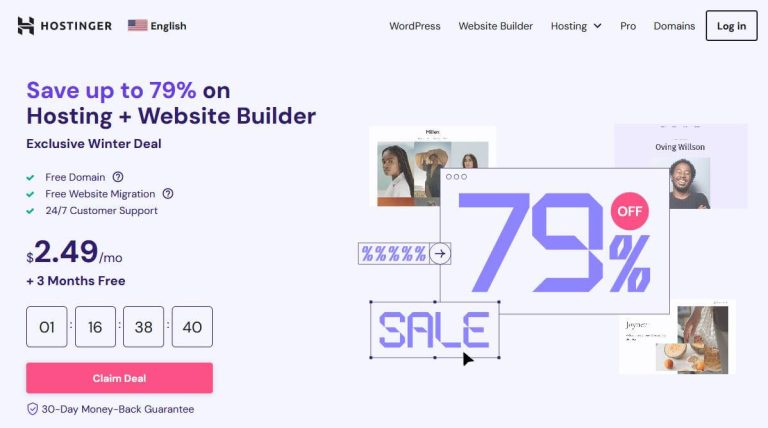This image captures the homepage of Hostinger's website, with a focus on their exclusive winter deal. The image is in landscape format, presenting a wide view. 

In the top left corner, the Hostinger logo is displayed, consisting of an 'H' formed by combining a lowercase 'n' and an uppercase 'N'. Next to the logo, "Hostinger" is written in black capital letters. Adjacent to this, an American flag icon followed by the word "English" in black is visible.

Continuing along the top menu, there are options listed as "WordPress", "Website Builder", and "Hosting" with a downward arrow, "Pro Domains", and "Login" highlighted in a black outlined box.

On the left side of the image, bold purple text advertises savings of up to 79%, followed by blue text mentioning "on hosting and website builder" beneath a banner that reads "Exclusive Winter Deal". Below this, three green check marks list benefits in small gray text: "Free Domain" with a question mark icon, "Free Website Migration" with a similar icon, and "24/7 Customer Support". 

Under the benefits, the price of $2.49 per month is announced, with an additional note of "plus 3 months free". Below this, a countdown timer is displayed, segmented into four boxes showing "01:16:38:40". A prominent pink button labeled "Claim Deal" in white text invites action.

At the bottom left, a shield icon with a tick mark assures a "30-Day Money-Back Guarantee". On the right side, five small square images are partially visible, with the central image displaying "79%" in large purple font, a pink circle with "OFF" in white letters above it, and the word "SALE" in stylized purple computer-like font with a grey outline and an arrow.

Background elements include subtle images: a photo of food that appears akin to wedding catering, the name "Oving Wilson" with a photo of a smiling black man in the top right, and the word "Milan" with photos of three women of diverse ethnicities in the top left, suggesting fashion-related content.